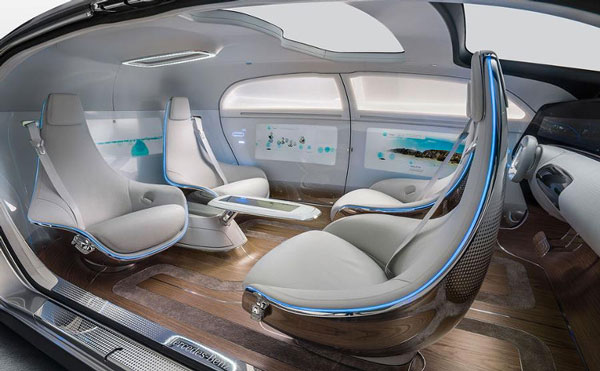This photograph depicts the interior of a highly futuristic and modern-looking vehicle, possibly a display model from Mercedes-Benz, as indicated by the branding. The vehicle's design is split open, likely for better exhibition of its advanced features. There are four very modernistic, high-tech bucket seats arranged in two rows facing each other, with metal frames enveloping their rounded, cushioned gray form. The seats, equipped with neon blue lighting accents and seat belts, exude a spacious and ergonomic design. The floor is an elegant hardwood, with a large sunroof above showering natural light into the space. The side paneling features high-tech graphics and even a map, enhancing the vehicle's futuristic appeal. The vehicle’s walls are a harmonious blend of shades of gray, white trim, and subtle hints of blue. A small table, extending out from a console between the rear seats, adds a practical touch to the innovative environment. The interior also includes a visible dashboard and steering wheel area, further illustrating the car's comprehensive, cutting-edge design.